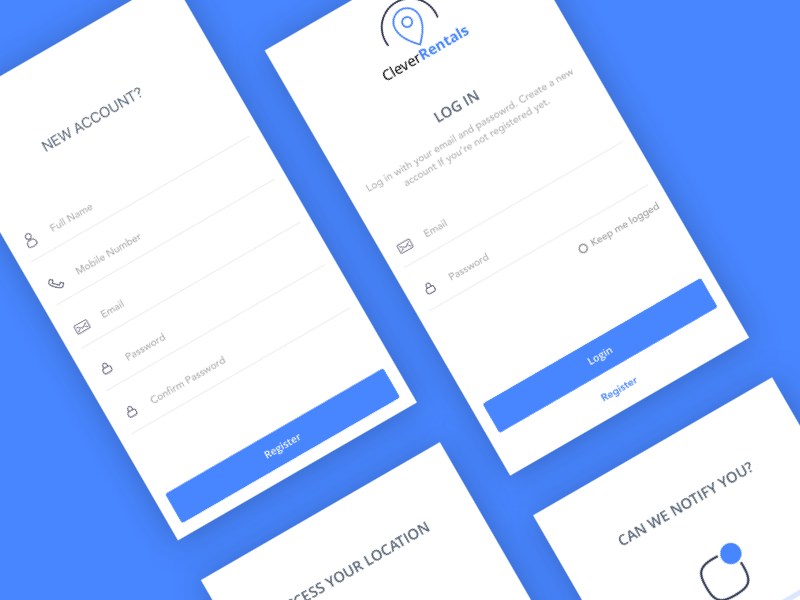The image portrays an arrangement of multiple smartphone screens diagonally aligned from the top left to the bottom right, showcasing various user interfaces of an application named “Clever Rentals.” The first screen displays a user registration interface where new users can enter their name, mobile number, email, password, and confirm their password. A prominent blue button for account registration is situated at the bottom of this screen.

The second screen features the Clever Rentals logo, resembling a light bulb with an arch above it, positioned at the top. Below the logo is a login interface where previously registered users can input their email address and password. An optional 'keep me logged in' checkbox is also available, along with a login button beneath it. For those who have yet to register, a conveniently placed 'register' button is located on the same screen.

The subsequent screens provide a glimpse into additional app features. One screen partially shows a prompt asking for location access, while another partially reveals a notification setup screen allowing users to enable notifications. Both screens only partially render, suggesting further functionality within the app.